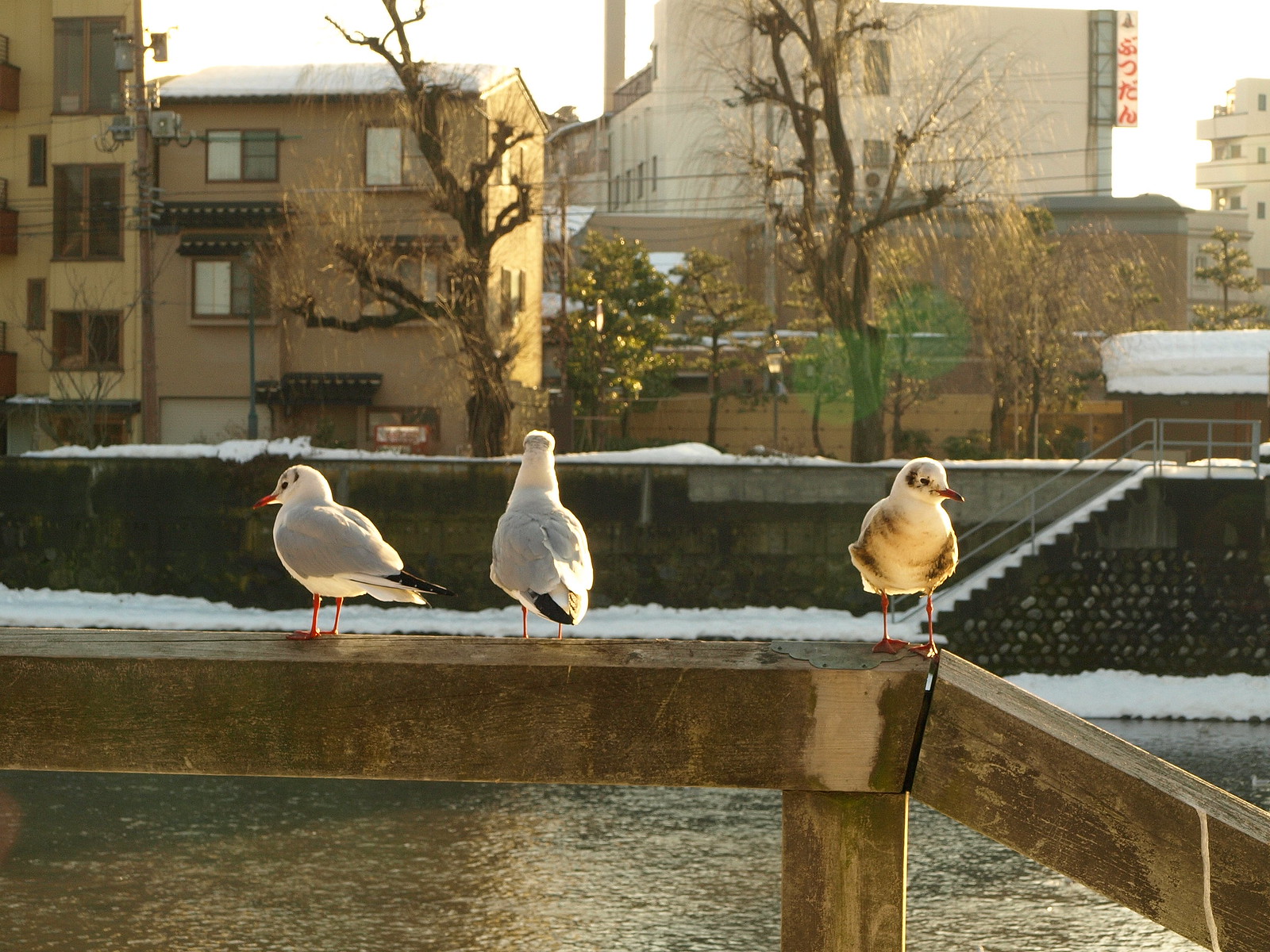A detailed photograph captures a wintry scene by the edge of a canal. The central focus reveals a worn, weathered wooden railing dusted with snow, where three birds, resembling seagulls, are perched. One bird faces the camera, one is in profile facing left, and the third looks away across the canal. Below, the water shimmers with reflections, tinged in brownish-gray hues. On the far side of the canal, a snow-covered concrete wall rises, featuring steps that lead up its surface. Beyond the canal, a backdrop of brown, brick apartment buildings with numerous windows is visible, framed by barren, leafless trees. The scene is illuminated by a subdued winter sun under a blue sky, contributing to the crisp, serene ambiance. Additionally, an adjacent rock holds a small cluster of pebbles, partially concealed by snow, further emphasizing the wintry atmosphere of the image.